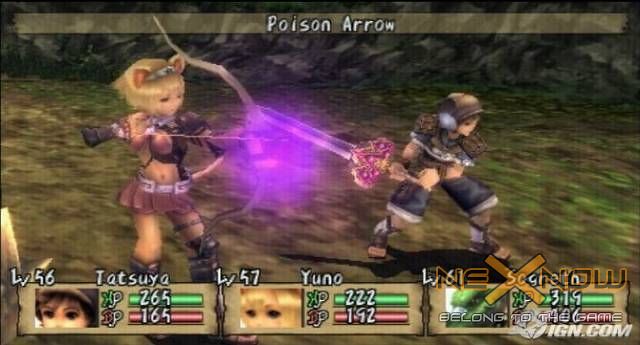This detailed screen capture from a fantasy fighting game, which resembles styles like Tekken and Street Fighter, features two elf-like characters with anime-inspired designs. The frame, which is horizontally rectangular, shows a somewhat grainy greenish land as the background. At the top of the screen, a banner with white lettering spells out "Poison Arrow." In the center, the blonde female character named Yuno, at level 57, readies a bow and arrow aimed at her opponent. Facing her is the male character Tatsuya, at level 56, wielding a giant sword to deflect Yuno's attack. Their point of contact is illuminated in neon purple. Along the bottom edge, there are three horizontally rectangular boxes displaying character statistics, including experience points (XP) and another scoring metric (IP). Another character, Sorath, is mentioned behind the screen capture logo, listed as level 61. Overall, this image captures an intense moment in a colorful, anime-styled fantasy battle.